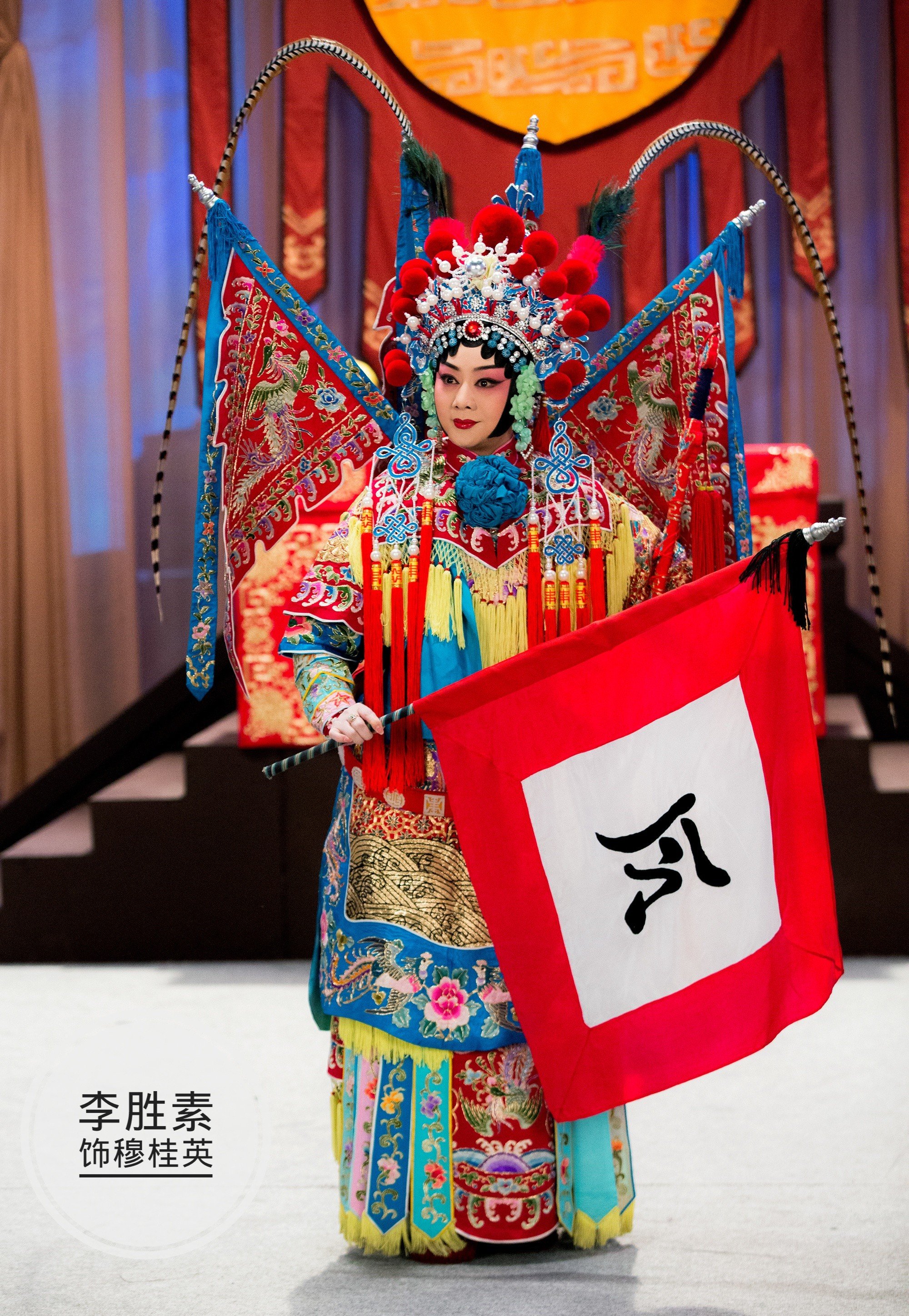The image depicts a Chinese opera singer standing on stage before a backdrop of black stairs and curtains. Central to the background is an orange tapestry flanked by red banners. She is adorned in a highly ornate, traditional costume, lavishly embroidered with an array of vibrant colors including pink, blue, turquoise, and red. Her elaborate headpiece features numerous intricate details such as little balls, large pearls, beads, jewels, and prominent red balls perched atop her head. Side pieces with fringe tassels dangle alongside her face. She wears dramatic stage makeup, with a white base, red accents around her eyes, and bold black outlining, complemented by red lipstick and thick eyebrows. From her back, poles extend to support large flags, embellished with red and blue hues as well as dragon motifs. Draping over her shoulders are red and yellow threads featuring floral patterns. She holds a flag marked with a Chinese character, and a second red flag bearing a white square with another symbol. Her attire and the presentation combine to form a vibrant and harmonious display of traditional Chinese opera aesthetics.